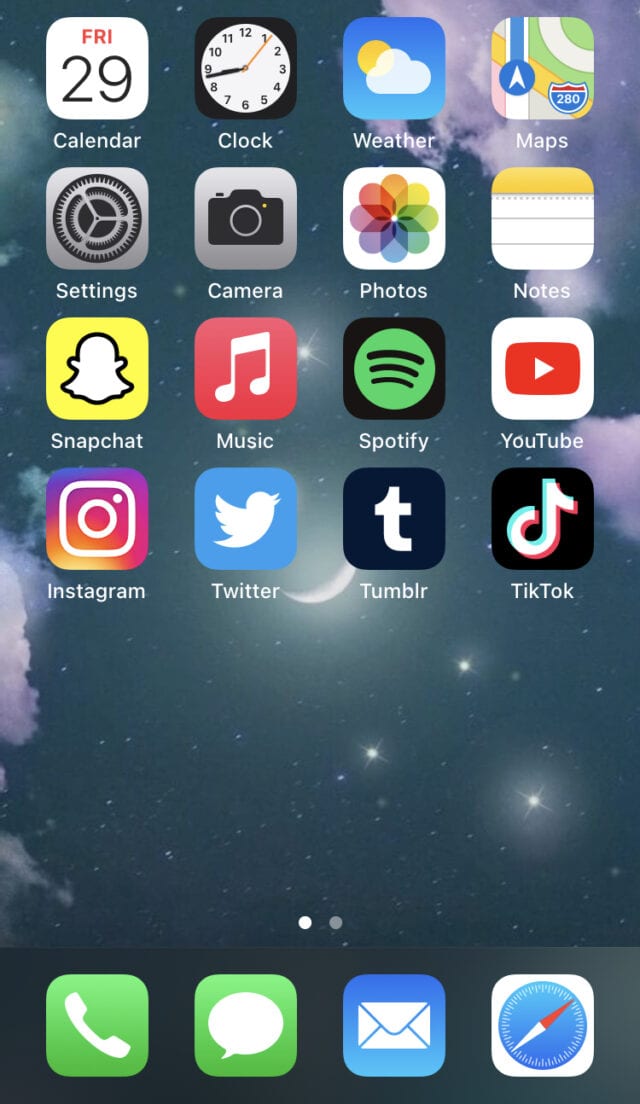This image is a detailed screenshot of the home screen of an iPhone. The screen features a total of 20 app icons, distributed with 16 on the main screen and 4 docked at the bottom. The icons in the dock, identifiable by their images, are Phone, Messages, Mail, and Safari, although these icons lack visible labels.

The home screen is on the first page, as indicated by two small circles at the bottom, with the leftmost circle filled in white, showing it is selected. 

The visible apps, arranged from the top left to the bottom right, are as follows:
1. Calendar
2. Clock
3. Weather
4. Maps
5. Settings
6. Camera
7. Photos
8. Notes
9. Snapchat
10. Music
11. Spotify
12. YouTube
13. Instagram
14. Twitter
15. Tumblr
16. TikTok

Each app icon is accompanied by a label displaying its name.

The background image of the home screen is a serene starry night sky, featuring a few clouds, a crescent moon, and several prominent stars, contributing to the peaceful aesthetic of the screen.